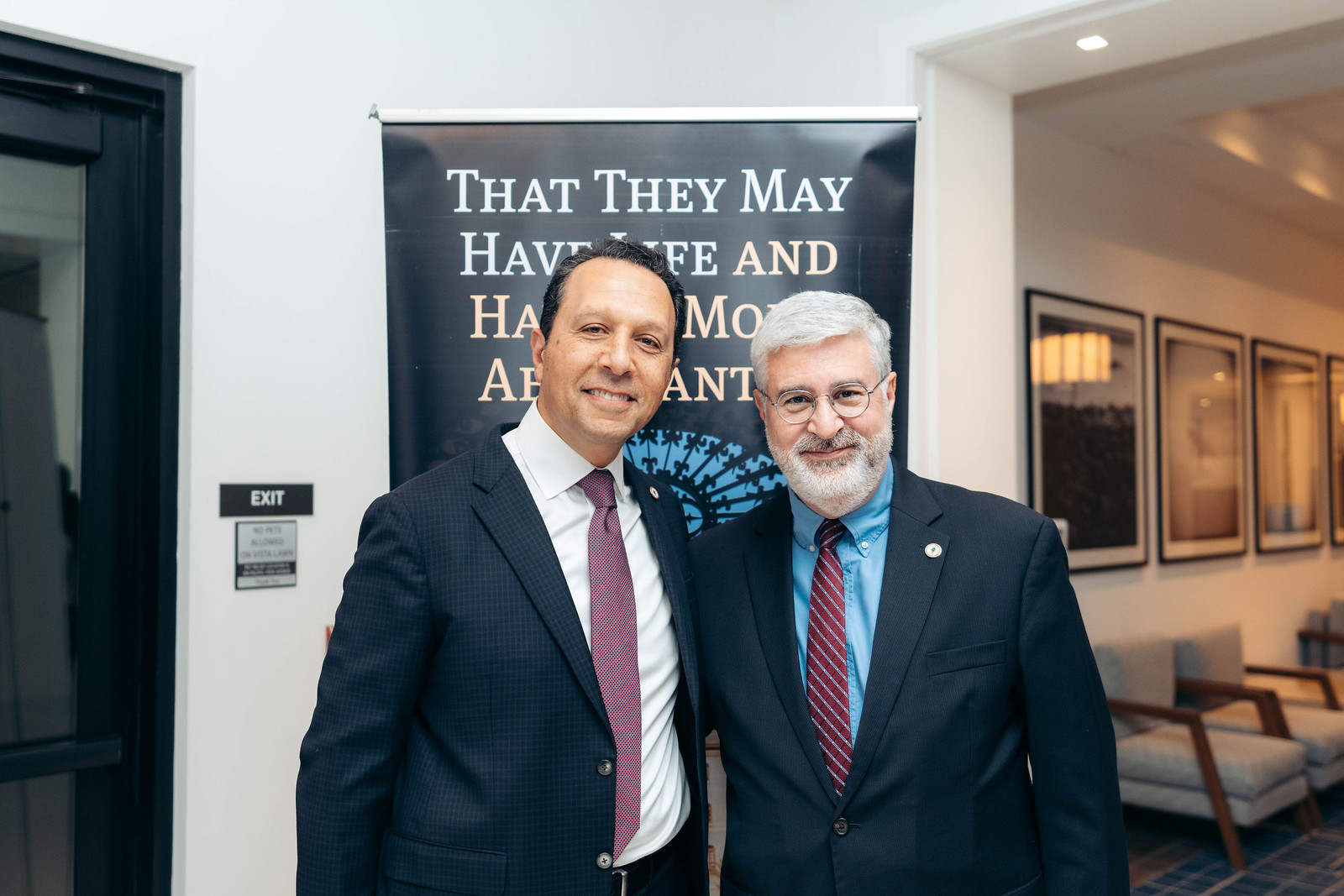This photograph, taken indoors in an office-like setting, captures two men standing side-by-side with their arms around each other, smiling at the camera. On the left is a man with short dark hair, possibly a white or Latino male, dressed in a black suit and a purple tie. To his right stands an older white male with gray hair, a gray beard, and a gray mustache, wearing eyeglasses, a navy blue suit, a red tie, and a blue button-down collared shirt. Behind them is a white wall adorned with a framed sign that reads, "They that may have life and have it more abundantly." Additionally, a doorway on the right side of the image leads to a waiting or reception area furnished with chairs and framed pictures on the white walls.